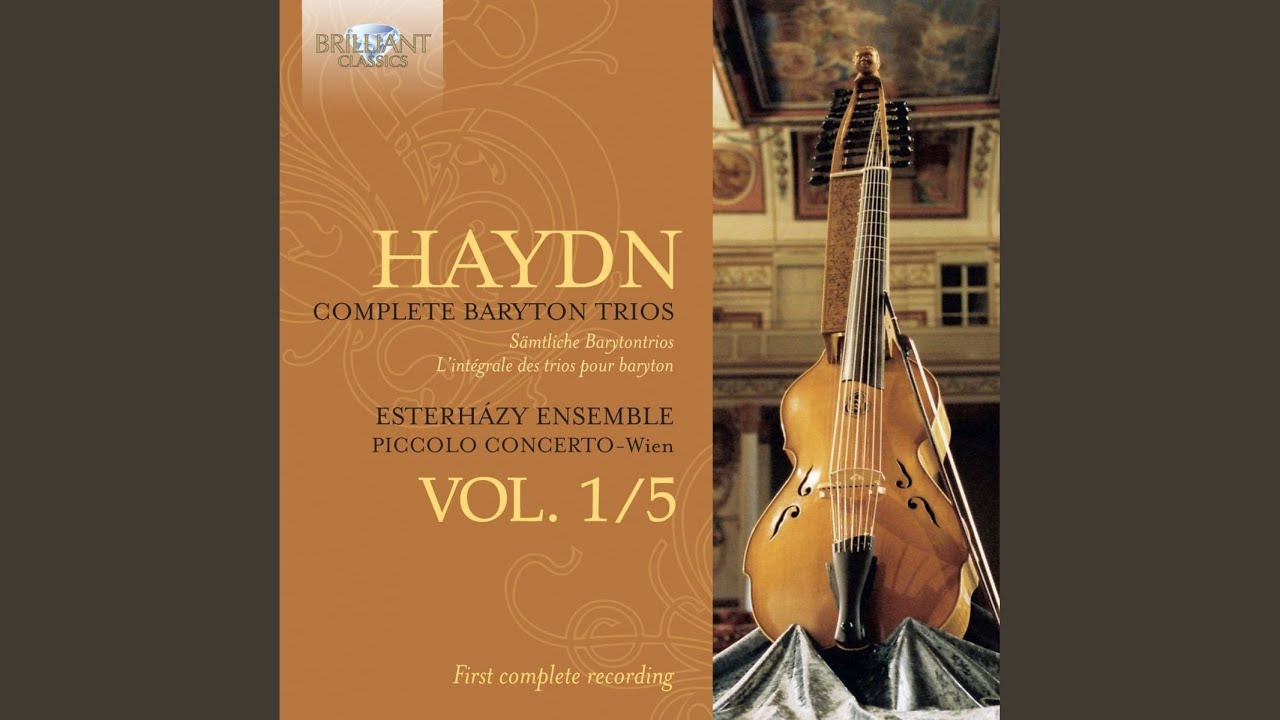The image appears to be a cover for a CD or a collection of music, featuring a dark brown-gray background. On the left side, there's a lighter brown rectangle with a diamond emblem at the top, above the text "Brilliant Classics." The central focus is on the title "Haydn" in large yellow font, and beneath it, "Complete Baritone Trios" in dark font. This is followed by multi-lingual text, including “Semtlick Baritone Trios” and “Le Tengral de Trios pour Baritone” in yellow.

Further down, the text includes "Esterházy Ensemble Piccolo Concerto Wien" in black, and "Volume 1 out of 5" in yellow. At the very bottom, it reads "First Complete Recording."

To the right of the text is a photograph of a baritone, a stringed instrument similar to a cello but with seven or eight strings. The baritone is pictured standing upright with a beige, gold, and cream color scheme, placed against a richly decorated, baroque-style background with frescoes and murals. The instrument is resting on a surface draped with black cloth.